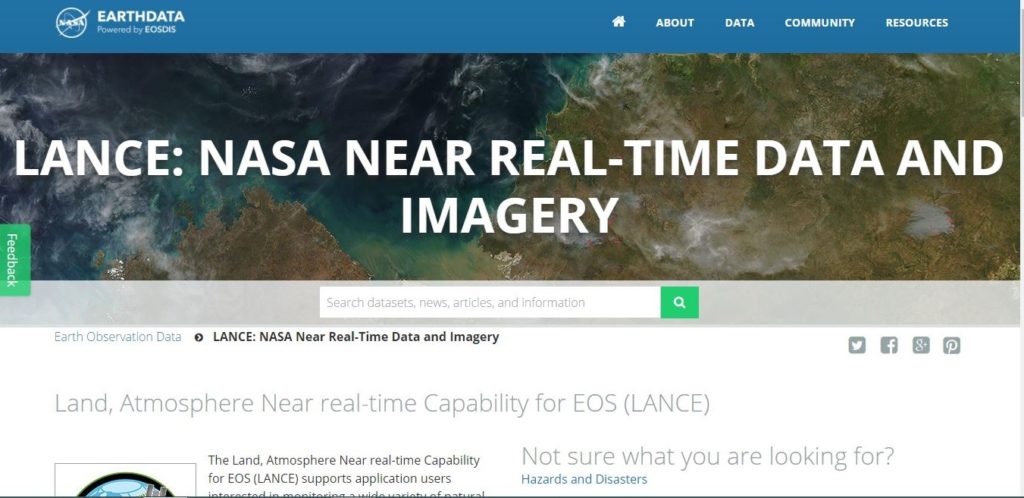Screenshot from the NASA Earth Data Site showcasing its capabilities. The blue header at the top displays "Powered by EOSDIS", accompanied by navigation options: Home, About, Data, Community, and Resources on the right. Dominating the page is a detailed satellite image from space, featuring water bodies, arid shorelines, and scattered clouds. Overlaying this hero image, bold white capital letters announce: "LANCE: NASA Near Real-Time Data and Imagery". 

On the left edge, a green feedback tab is visible, and beneath the hero image is a gray bar featuring a search field labeled "Search datasets, news articles, and information", with a adjacent green search button. Below this, "Earth Observation Data, LANCE, NASA Near Real-Time Data and Imagery" is prominently displayed in black text. 

To the right, under the gray search bar, are social media icons for Twitter, Facebook, Google+, and Pinterest. Further down, light gray text spells out "Land Atmosphere Near Real-Time Capability for EOS LANCE". 

To the lower right, the options include a section named "Hazards and Disasters", partially obscured by a cut-off icon and text. The bottom of the page is framed by another gray bar.